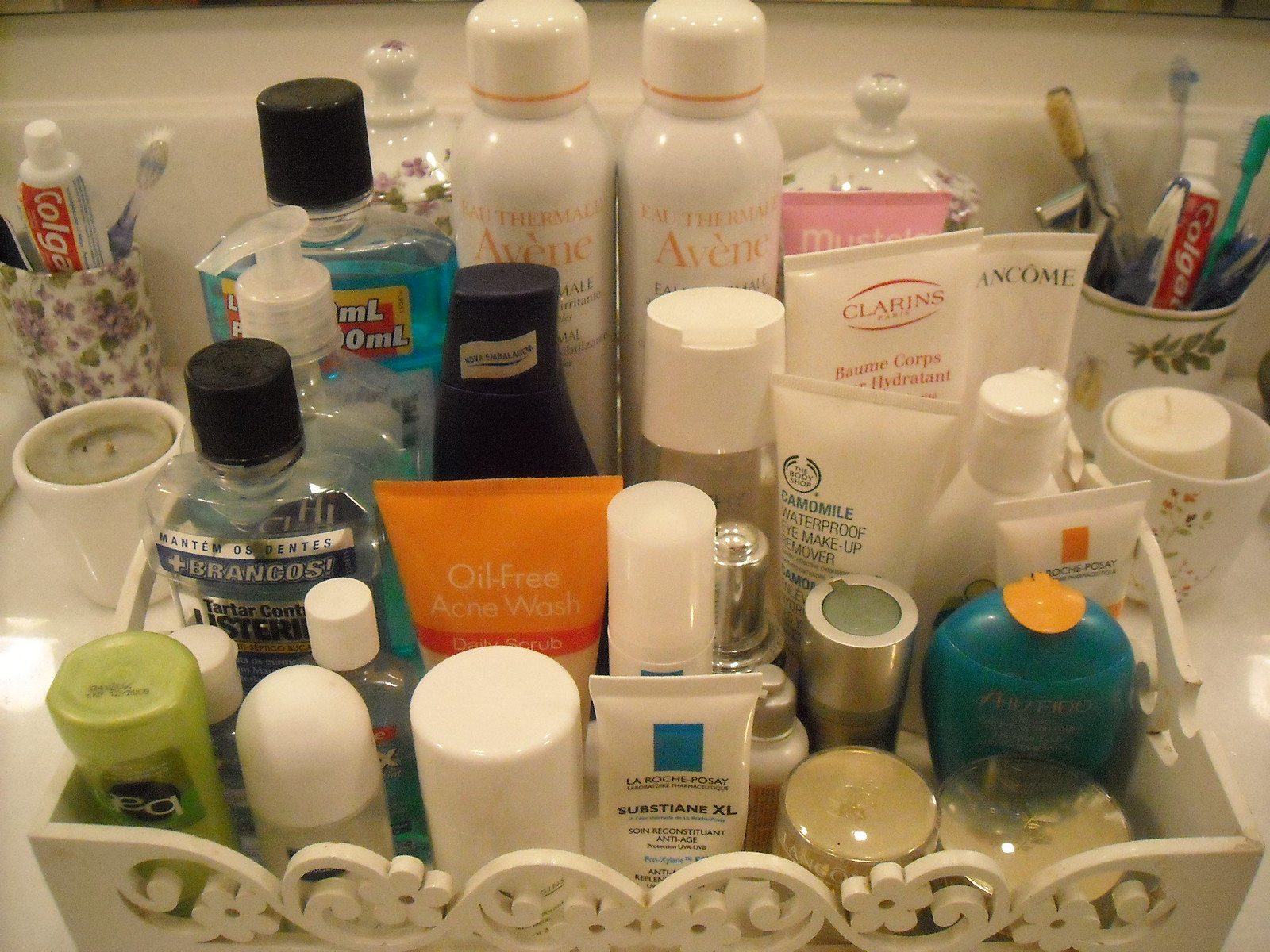In this photograph, a variety of beauty, skincare, and health products are neatly arranged on a gleaming white, glossy-finished bathroom countertop. Central to the display is a decorative white wooden box adorned with a floral design and a waved pattern, holding an assortment of containers.

Towards the back of the box, a mouthwash container filled with blue liquid and sealed with a black cap is partially visible. Next to it stands a bottle of Listerine marked "Tartar Control." Nearby, a hand soap dispenser is placed prominently along with several smaller bottles with white caps, likely hand sanitizers. The box also holds a small green container and several white-lidded containers resembling deodorants.

To the right, a collection of taller cream-colored tubes, possibly moisturizers, makeup removers, or facial cleansers, adds to the array. A teal shampoo bottle with an orange lid is also seen among the assortment.

Framing the scene, the background features two white ceramic cups, each housing a candle — a green candle on the left and a white one on the right. Additionally, two floral print ceramic containers flanking the arrangement hold various personal care items, such as razors, toothbrushes, and toothpaste, completing the organized yet visually appealing setup.